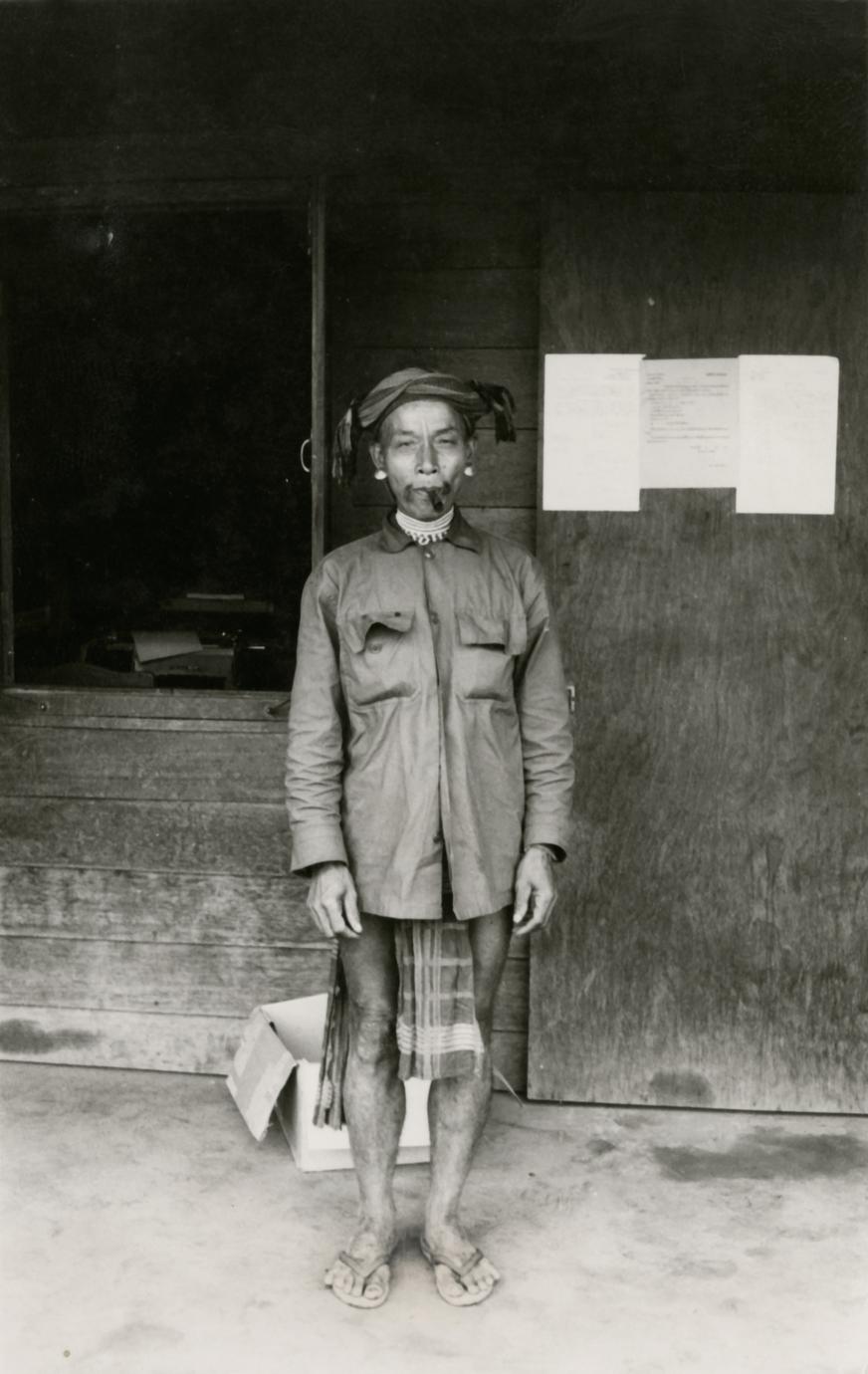This detailed, consolidated caption offers a comprehensive description of the black-and-white photograph by merging shared and emphasized details from each of the three original captions:

"This black-and-white photograph, seemingly taken in the early 1900s, features an older man, possibly of indigenous Maori heritage. The man stands in front of a wooden building, beside a wooden door with stapled white papers and beside an open doorway. His outfit includes a distinctive moon-shaped leather jacket, a headwrap or turban, and earrings. He has a stern expression with a hint of a mustache and possibly a tattoo beneath his lower lip. A cigar or blunt hangs from his mouth, and he is barefoot except for sandals. Behind him, a cardboard box and a possible typewriter can be seen through a nearby window. The surrounding setting includes steps leading up to the doorway and various indistinguishable items scattered on the floor."